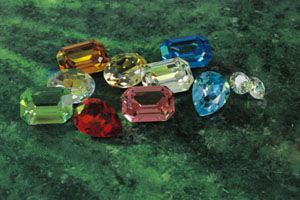The color photograph showcases an array of 11 meticulously arranged gemstones, displayed on a luxurious emerald green fabric that appears exceptionally soft. The collection includes prominent gems such as a diamond, an emerald, a sapphire, and a ruby. Among these are also a yellow topaz and a delicate pink stone, alongside additional smaller diamonds likely cut for rings or earrings. The stones vary in shape and cut, featuring traditional round, teardrop, square, and rectangular faces. Each gemstone is polished to perfection, radiating clarity and brilliance, with some exhibiting a birthstone-like quality. The overall presentation highlights the exquisite craftsmanship and beauty of the jewels, set against the rich green backdrop.